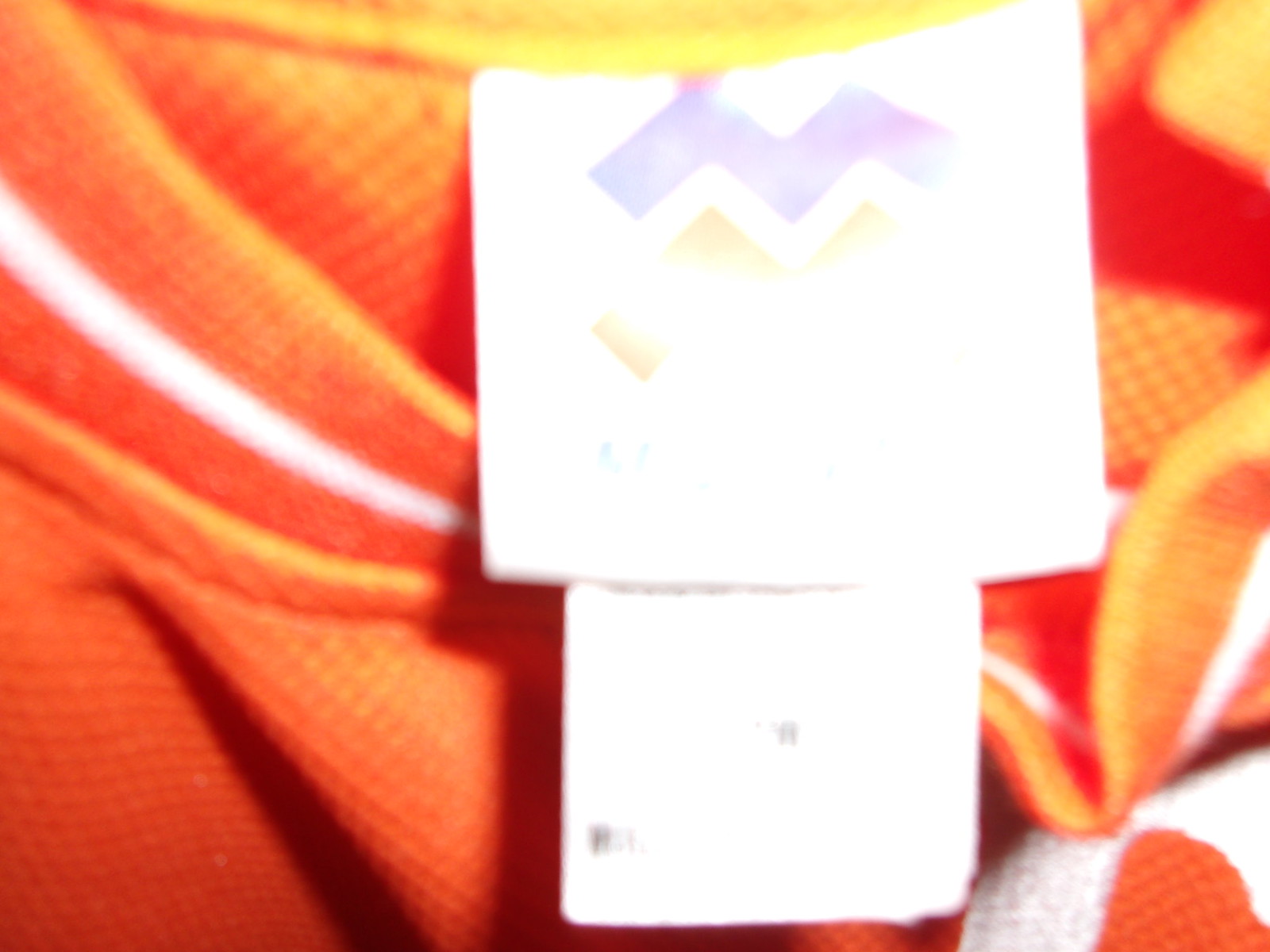The photograph depicts an orange shirt neatly folded, with its label prominently sticking out. Due to overexposure, the lighting distorts the image, making the label appear intensely white and obscuring the logo and other text details. The label features a main section and a secondary tag providing size and washing instructions. The shirt's collar is rimmed with stripes of orange, white, and a golden-yellow hue, adding a distinctive touch to its design. Due to the lighting, specific markings on the label remain indistinguishable.